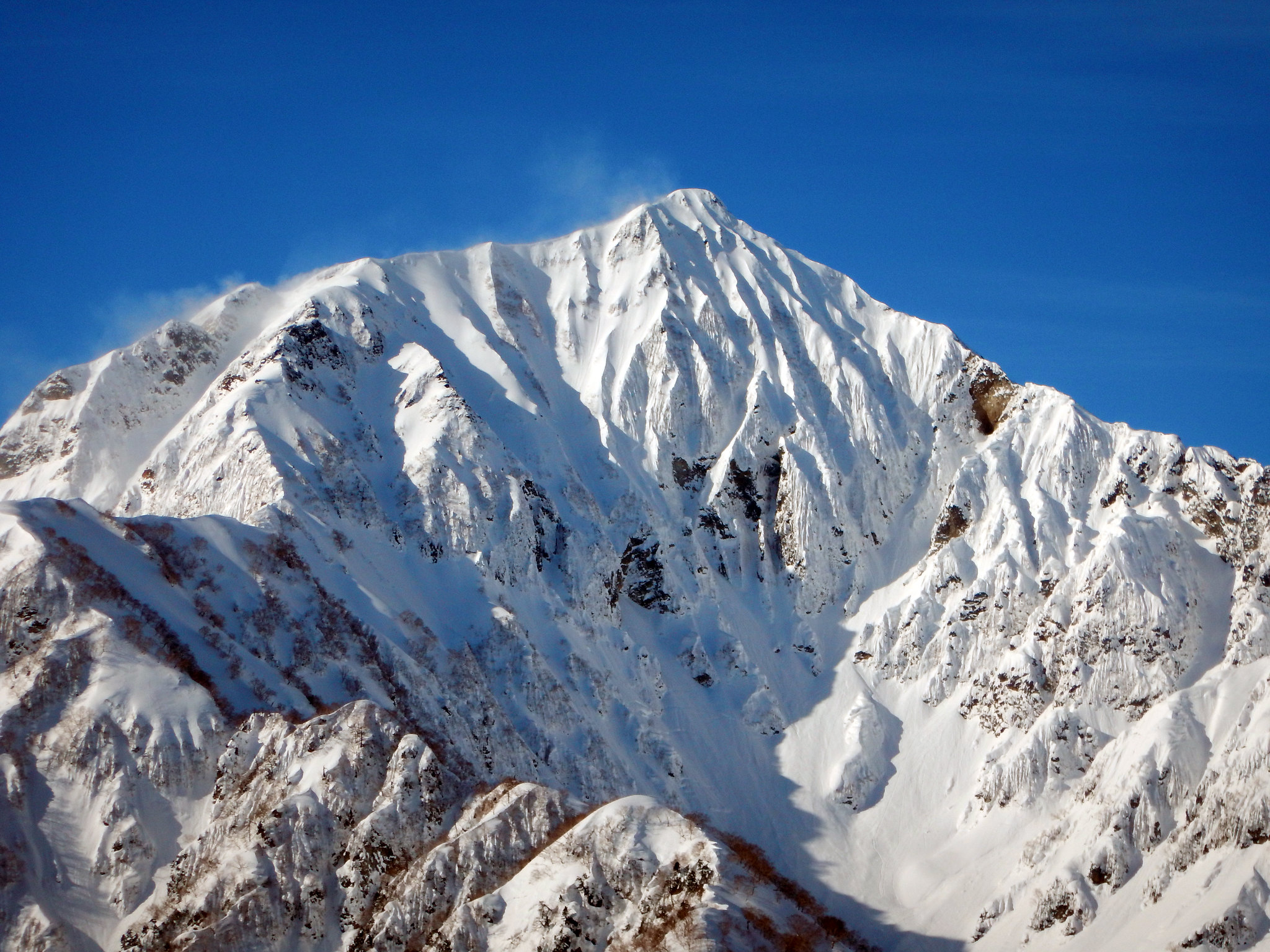A stunning daytime scene of a snow-capped mountain range bathed in natural sunlight under a bright blue sky. The snow-covered peaks dominate the image, showcasing their pristine white beauty. In the bottom left-hand corner, the lower part of the range is visible, with trees poking through the snow, giving a reddish-brown hue to the landscape. This reddish-brown hue continues to be visible in the lower portions of the mountain on the left side. As we move to the middle left of the image, strong layers of snow intermingle with the reddish hue of the trees, this area covered in shade. At the very top of the mountain, wisps of what appear to be clouds, smoke, or mist drift off the peak, adding a sense of mystique. The central part of the mountain is shaded, accentuating the contrast between light and shadow. On the right-hand side, a brown patch of the mountain surface is exposed where the snow has not settled or has fallen off, further highlighting the mountain's varied texture and color.